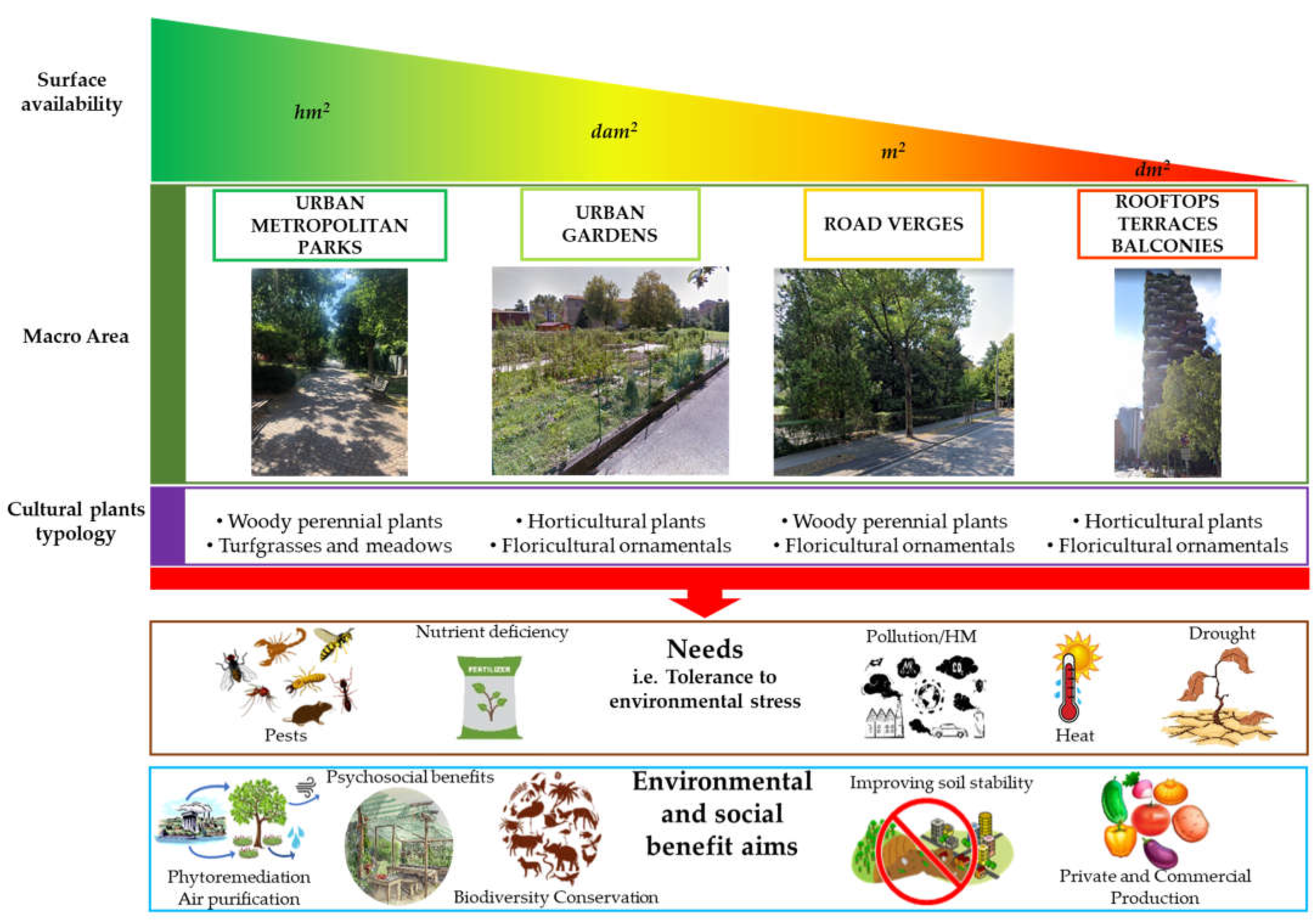This poster serves as an environmental educational piece detailing the types of plants suitable for various urban areas, their specific needs, and associated environmental and social benefits. At the top, a gradient chart starting from green on the left and transitioning through yellow and orange to red on the right, delineates surface availability. It begins with urban metropolitan parks in green (HM2), followed by urban gardens in yellow (DAM2), road verges in orange (M2), and ends with rooftop terraces and balconies in red (DM2).

On the left of this chart, labels for macro areas describe different urban spaces. The black-text categories indicate the types of vegetation: urban parks support woody perennial plants, turfgrasses, and meadows, while urban gardens mostly contain horticultural plants. Road verges host woody perennial plants and floricultural ornamentals, whereas rooftops, balconies, and terraces contain both horticultural and floricultural plants.

Below this gradient chart, another detailed block labeled "Needs" outlines environmental stress tolerance requirements. These include pests, nutrient deficiencies (depicted with a bag of fertilizer), pollution (represented by dark clouds and factory smoke), temperature extremes (indicated by a red temperature gauge), and drought conditions (illustrated with a dead, arid-plant image).

At the bottom of the poster, there is a blue rectangular block titled "Environmental and Social Benefit Aims." This section highlights the ecological advantages of urban greenery like biodiversity conservation, soil stability improvement, air purification, and psychosocial benefits. Visual illustrations accompany these descriptions, such as a cityscape emphasizing air purification and a group of vegetables symbolizing private and commercial production.

Through detailed charts, illustrations, and explanations, this poster effectively communicates the variety of plants suited to different urban environments, their specific needs, and their multifaceted benefits.